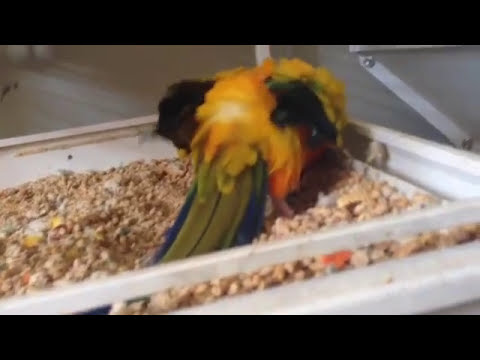The image depicts a small bird, likely a parrot or cockatoo, viewed from the back inside a non-typical white bird cage situated in a room with a hardwood floor. The bird's plumage is mostly golden yellow, with some black or dark navy blue feathers on its wings. Its tail feathers are a vibrant mix of green, blue, and slightly olive green in the middle. The bird is bent over, seemingly engaged in eating from the cage floor, which is covered in a rough, brown, Rice Krispie-like material or tan-colored gravel with some yellow and orange bits. The cage itself features a screen or clear plastic between white-framed sections, adding to its unique look. The bird's head is not visible, as it appears to be burying it into the feeding material.